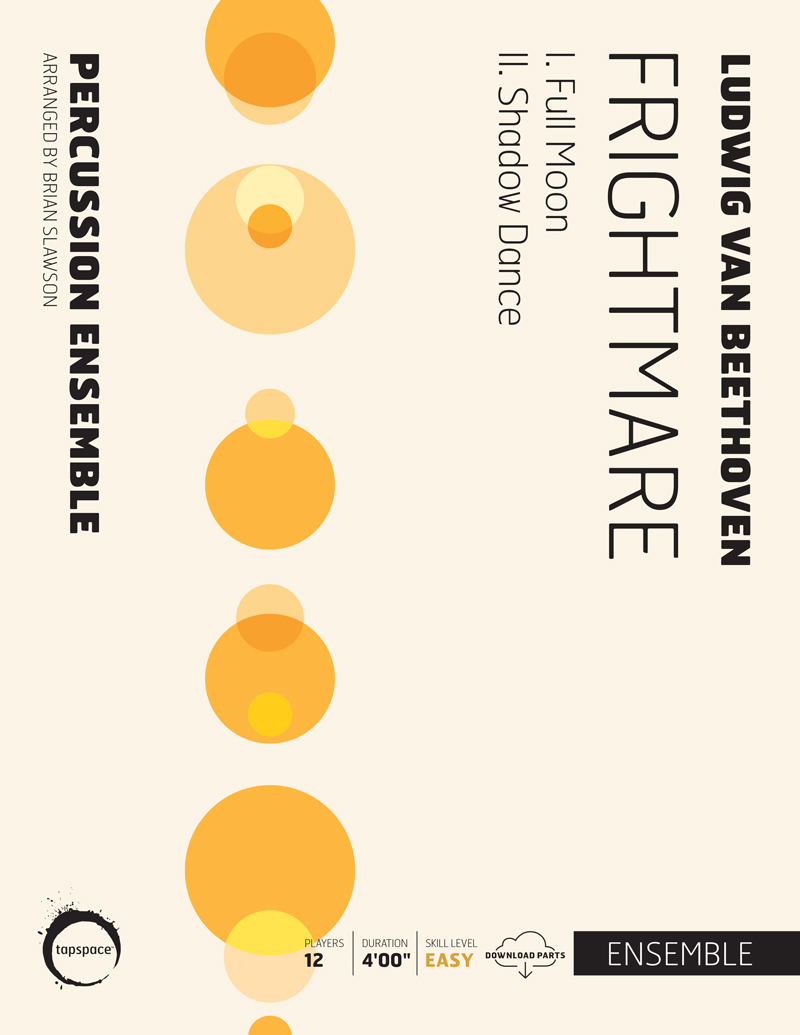This intricate image, likely promotional artwork for an event or ticket, prominently mentions "Ludwig van Beethoven Frightmare: One Full Moon, Shadow Dance." Against a black background with variations from dark to light black, the central focus includes a series of yellow and orange geometric shapes, composed of larger circles interspersed with smaller ones, suggesting a rhythmic or bubble-like pattern.

Text is arranged in both vertical and horizontal orientations. Vertically aligned on the left, the text starts with "Ludwig van Beethoven," followed by "Frightmare," "One Full Moon," and "Shadow Dance." Horizontally across the base, it reads "Percussion Ensemble, arranged by Brian Slauson," highlighting the ensemble's role in the performance. In the bottom left corner, there is additional information: "Duration 4, Skill Level Easy," and "Players 12," next to the logo for a company named Cardspace. The section to the right includes text like "12 4 0 0" and the word "easy," along with a black block containing the word "ensemble" in white lettering, all contributing to the event's details.